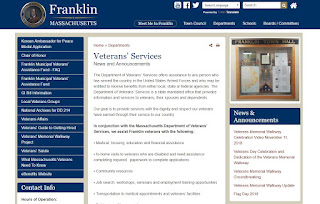Here's a carefully detailed and cleaned-up caption for the described image:

---

"The image, although small and blurry, appears to be a screenshot of the Franklin, Massachusetts, municipal website. The background predominantly features a clean, white color scheme complemented by dark blue accents. At the top, there is a large dark blue header or banner displaying 'Franklin, Massachusetts' on the left side alongside a small circle containing an image of an individual. Moving to the right side of this header, there appear to be several functional icons possibly for login or registration, a search bar, and a home button.

Below the header, there is a navigation menu with several options, although the text is too pixelated to be clearly read. Beneath this menu is a section with a sandy, beige background. To the left of this section is a sizable dark blue sidebar showcasing various options, potentially representing popular links or menu choices. Adjacent to this is a box containing contact information, but the details are illegible due to the blurriness of the image.

In the center of the page, there's a large white box labeled 'Veterans Service', though specifics about this service remain unreadable. On the right side of this central box is a smaller box with an image inside. Below these elements, another box is labeled 'News and Announcements' with several announcements listed underneath, though the text again remains too blurry to interpret."

---